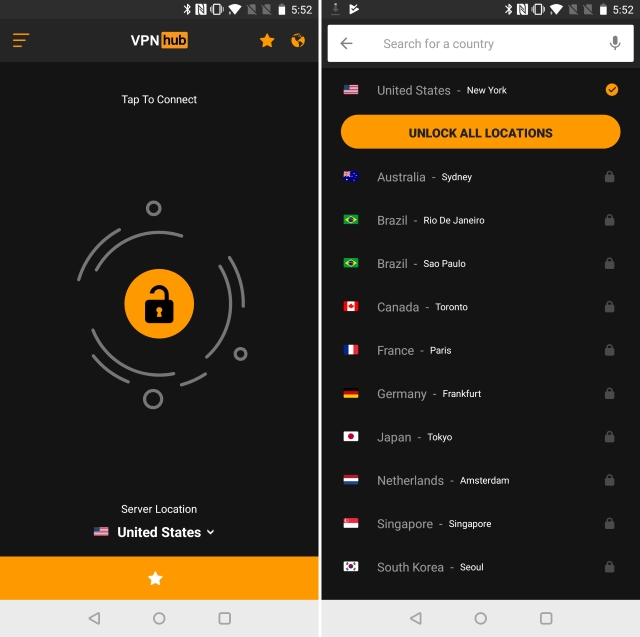The image showcases a side-by-side comparison of two screenshots from a VPN mobile application interface. The left screenshot prominently features a gold-colored, filled-in circle with a black, unlocked padlock icon in the center. Around this central icon are swirling lines, and the text "Server Location: United States" is displayed, accompanied by a US flag. Below this, an orange-gold button with a star reads "Tap to Connect."

In the screenshot on the right, the search bar at the top is empty. Directly below it, the location is set to "United States, New York." Beneath this, there is a long button labeled "Unlock All Locations." The list of alternative server locations includes various cities and countries: Sydney (Australia), Rio de Janeiro and Sao Paulo (Brazil), Toronto (Canada), Paris (France), Frankfurt (Germany), Tokyo (Japan), Amsterdam (Netherlands), Singapore, and Seoul (South Korea). This interface appears to allow users to switch their VPN connection between different international servers.